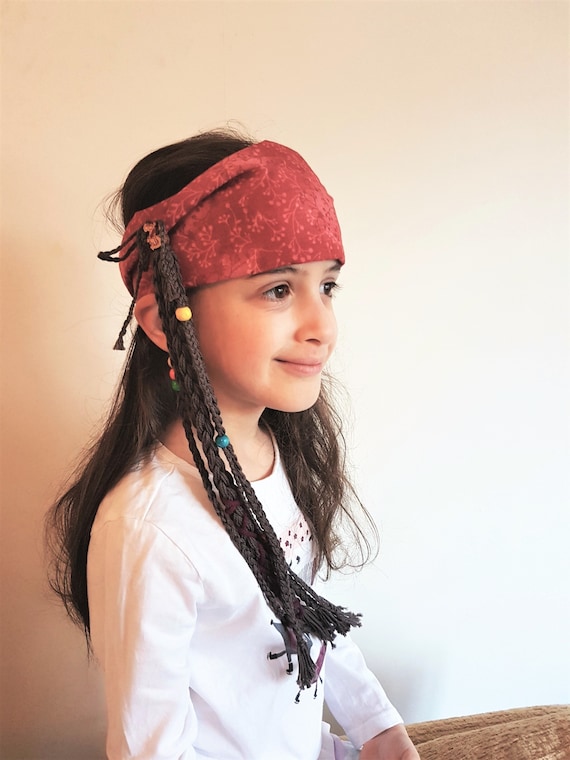This detailed, photographic-style indoor image presents a girl around eight or nine years old in profile, gazing from left to right. The girl has light skin, brown eyes, and long brown hair that is intricately styled. A red floral headband adorns her head, with tight braids peeking through a hole in the headband. Each braid is decorated with vibrant beads—yellow, blue, red, and green—that add a playful touch. She smiles gently, her pink lips forming a closed-mouth smile while her eyes sparkle with a hint of joy. Dressed in a white long-sleeved shirt patterned with polka dots, she stands out against a background that is lighter on the right side and shaded on the left and top edges. In the bottom right-hand corner of the photo, the edge of a brown sofa or furry beige cushion is faintly visible, adding a cozy element to the setting. The overall ambiance is warm and light-hearted.